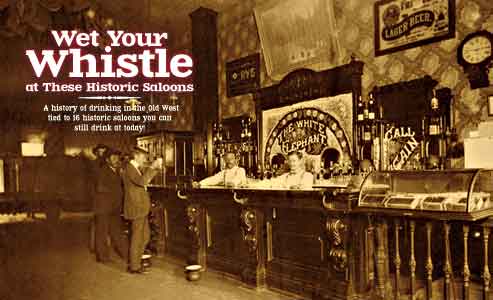A sepia-toned advertisement depicts a historic saloon, possibly from the 1930s or 1940s, with the text “Wet your whistle at these historic saloons” in white, framed by a glowing red border. Below this, it reads “A history of drinking in the Old West tied to 16 historic saloons you can still drink at today.” The saloon, named "The White Elephant," displays a sign that reads "lager beer" or possibly "lodger beer" and features a classic wall clock. Two Caucasian bartenders, dressed in white button-up shirts with bowties and suspenders, stand behind the bar. Three sharply dressed gentleman patrons are seen enjoying their drinks, adding to the nostalgic ambiance of the scene.